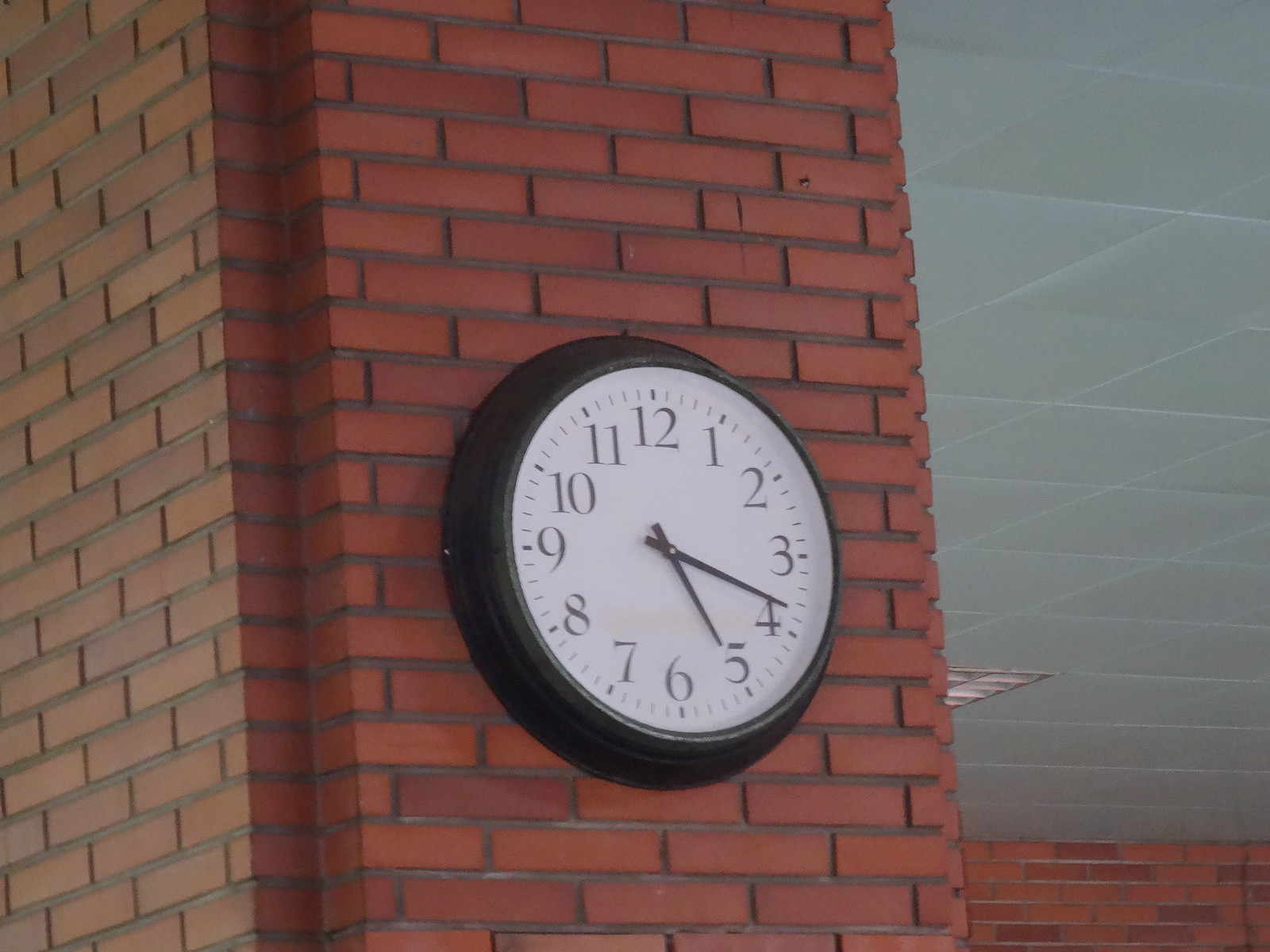In this photograph, the focal point is a wall clock mounted on a brick wall composed of dark burgundy and brown bricks, potentially indicating an exterior location, such as a library or school building. The clock itself features a white face with black numerical markings and slim, black minute and hour hands encased in a black border. To the right of the clock, there is a section of a white ceiling that merges with the same dark brickwork, creating a blend of textures and colors. Additionally, a white vent is visible towards the right side of the clock, attached to the ceiling, adding an element of utility to the composition. The environment's exact setting remains ambiguous, as it is unclear whether the scene is indoors or outdoors.